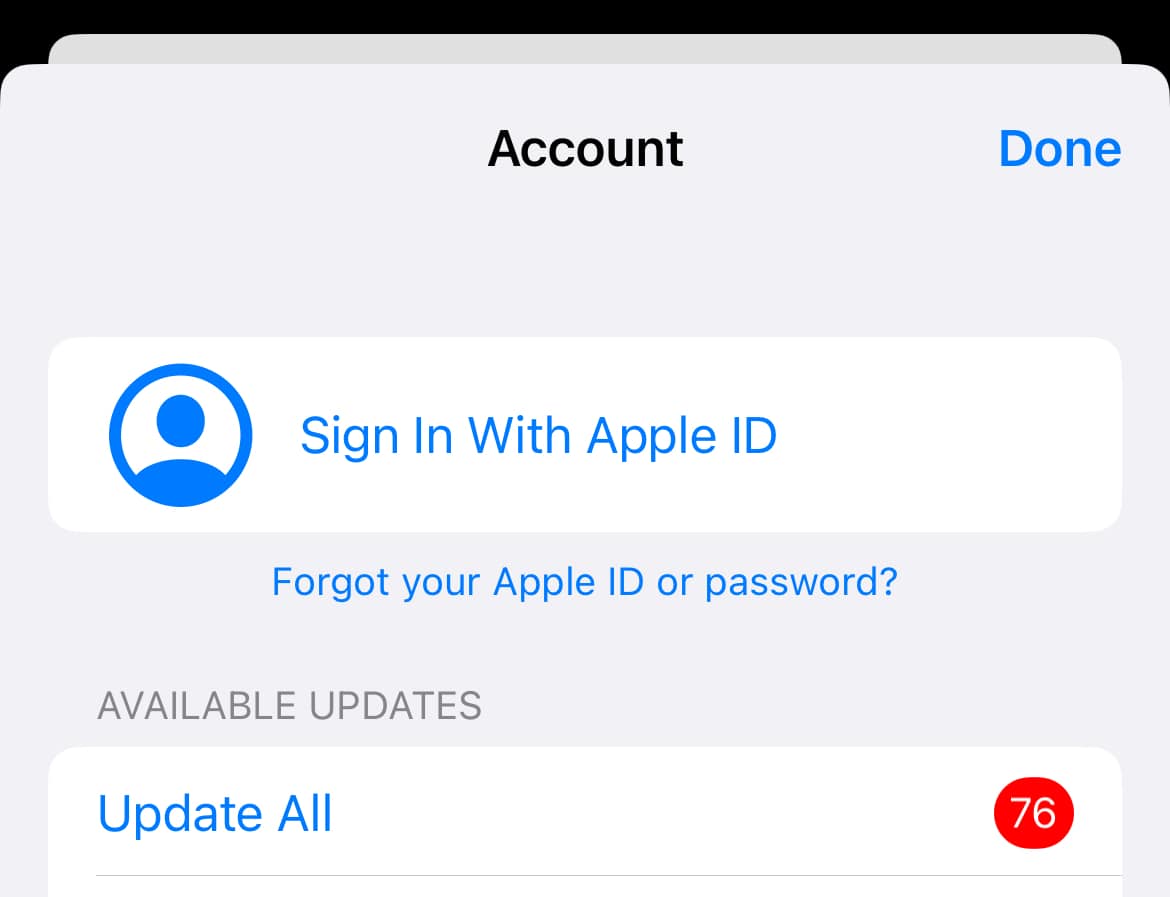Screenshot of an Apple ID Sign-In Page on a Mobile Device

The screenshot depicts a sign-in page for an Apple ID, displayed on what appears to be a phone or tablet. At the top of the page, against a black background, the word "Account" is centrally aligned in white text. In the upper right corner, there is a "Done" button, also in white text. Below, centrally positioned, there's a user icon depicted as a simplified figure with a head and shoulders inside a blue circle.

To the right of this icon, blue text reads "Sign in with Apple ID." Immediately below, there's a link stating "Forgot your Apple ID or Password?" in gray text. Further down, aligned to the left, the text "AVAILABLE UPDATES" appears in gray, capitalized letters. Adjacent to this, in blue text, is an "Update All" button, implying that there are software updates available.

A red badge with the number 76 in white is placed next to the "Update All" button, indicating the number of pending updates. This section is delineated with a simple gray line beneath it. The surrounding area of the page appears to have a simplified design, featuring a white curved area at the top, a predominantly black background, and a partially obscured gray button or field in the middle, hidden by the Apple ID sign-in overlay.

The overall design is minimalistic, focused on guiding the user to either sign in to their Apple ID or manage available updates.